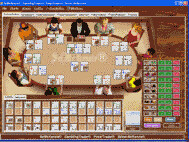A pixelated digital scene is presented in a very small image, which appears to be a screenshot from a browser window. The top of the image displays a classic blue browser bar with indistinguishable text on the left side and the minimize, expand, and close buttons on the right, with the close button highlighted in red.

Below the bar, the main focus is an 8-bit pixel graphic scene depicting approximately 10 characters seated around an oval table, seemingly engaged in a card game that could be blackjack, given that each participant has a pair of cards in front of them. The characters are dressed in varying attire, including a black suit, a gray suit, a red dress, and a yellow shirt, among others, creating a colorful and diverse group.

On the bottom right of the scene, a user interface (UI) panel features columns of green and red rectangles, possibly representing player statuses or game information. Just to the left of the UI panel, a grid of tiny, light brown squares along with unclear images, which may be additional cards or game elements, can be seen on the lower left side of the image. Despite the image's diminutive size, the vibrant pixel art adds a nostalgic charm to the intricate digital tableau.